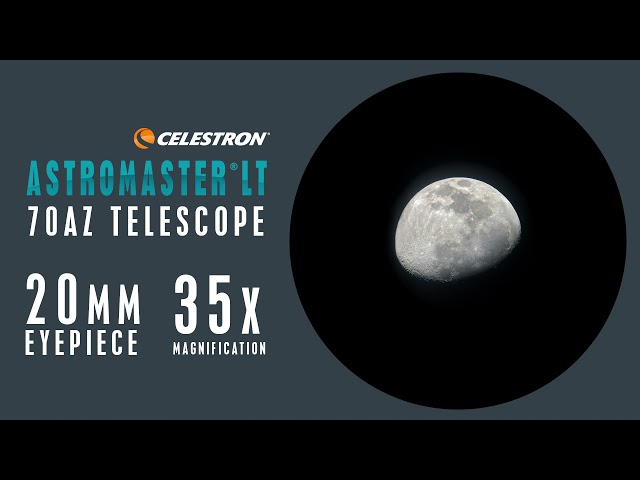This advertisement for the Celestron AstroMaster LT 70AZ telescope features a predominantly dark gray background with subtle blue shading, bordered by black bars on the top and bottom. On the upper left side, the orange Celestron logo, featuring a curved black line, is prominently displayed in white text. Below the logo, "AstroMaster LT," "70AZ Telescope," "20mm eyepiece," and "35x magnification" are clearly detailed in descending order. Dominating the right side, a large black circle showcases an image of the moon, which is light gray with white specks indicating meteor impacts and darker gray craters towards the top. This depiction aims to illustrate the visual clarity and magnified detail one can expect when using the telescope.